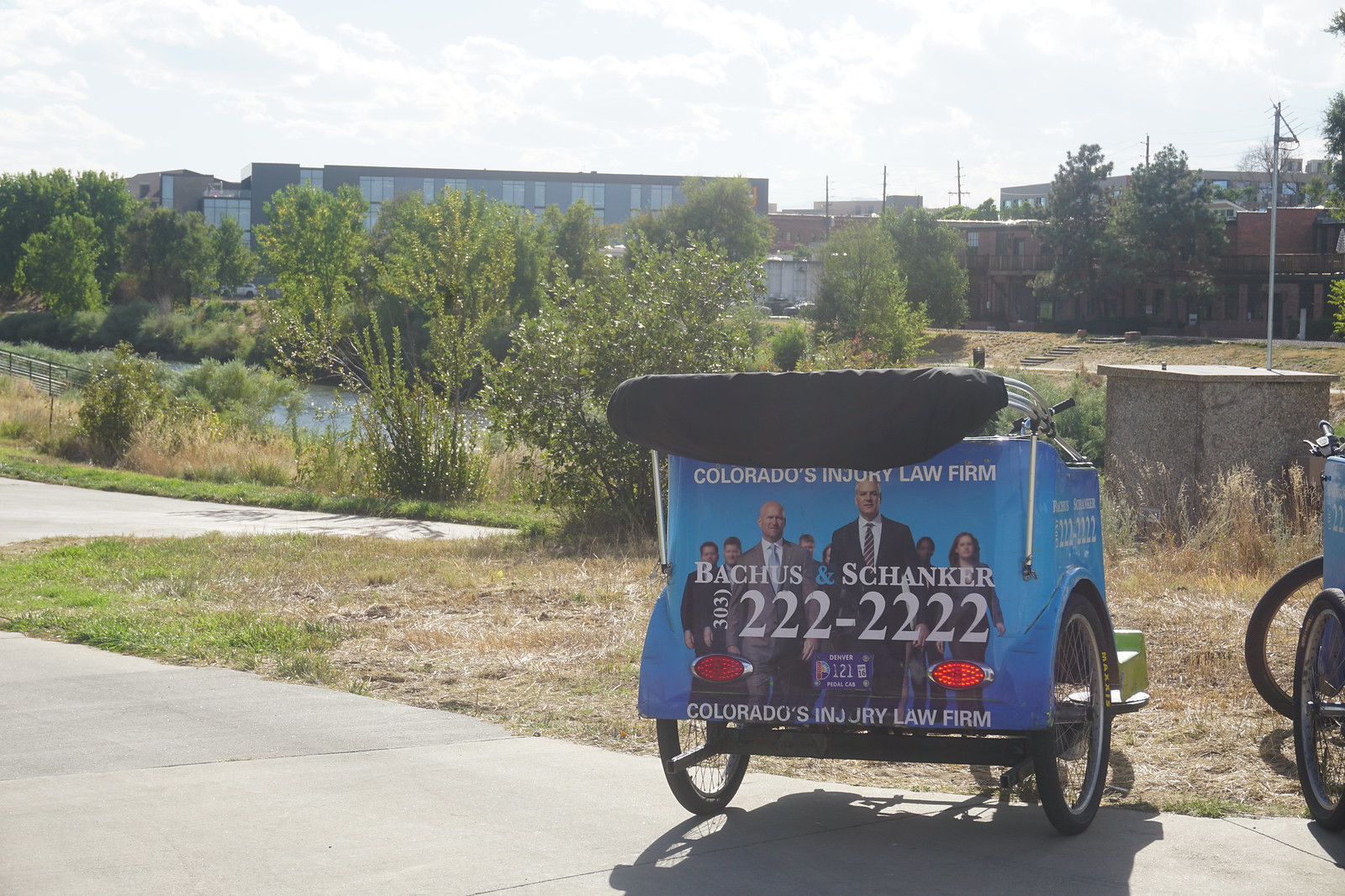The image depicts a blue rickshaw with black wheels, parked on a cement sidewalk against a backdrop of greenery. The rickshaw features a black cover that is currently down and an advertisement for "Colorado's Injury Law Firm" by Bacchus & Shanker, including their phone number, 303-222-2222. The ad prominently showcases several men and women in suits, likely the lawyers from the firm. In the background, there are green trees, a pond, and what appear to be apartment buildings under a bright, cloud-filled sky. Another similar cart is partially visible on the right. The setting includes a mix of dead and green grass, contributing to the vivid outdoor scene.